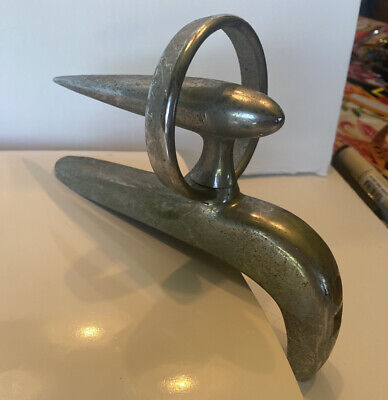The image depicts a vintage Ford bombsight hood ornament, a classic automotive decoration likely from the 1950s. The hood ornament is crafted from solid, strong metal, probably chrome, giving it a reflective sheen and a smooth surface. Central to the ornament is a torpedo-shaped figure that aligns horizontally, with its pointed end toward the back, encircled by a metal ring connected to the base stem. This base is cylindrical and curves gently to the right. Despite its aged appearance and signs of corrosion, the ornament retains its elegant design. The object is positioned on a beige, stair-like surface, with a white wall as the backdrop. To the right, there's a carpet-like area that features reddish and beige hues. The overall setting emphasizes the hood ornament's antique and historical significance.